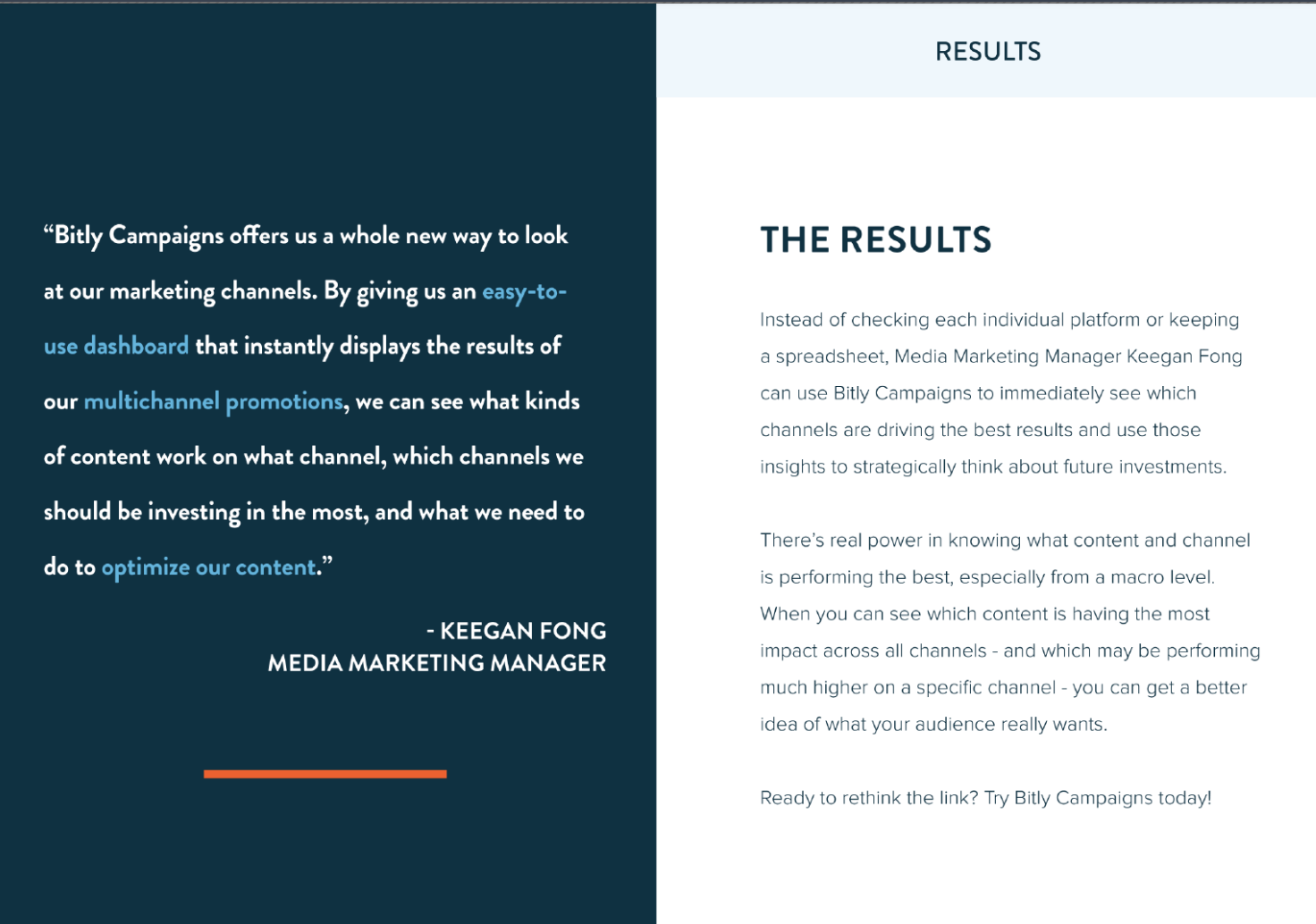The image is a promotional screenshot highlighting the benefits of Bitly Campaigns for media marketing. On the left side, there's a testimonial from Keegan Fong, Media Marketing Manager, explaining how Bitly Campaigns provides a comprehensive and user-friendly dashboard that displays the results of multi-channel promotions instantly. This allows users to identify which types of content perform best on specific channels, determine the most effective platforms for investment, and optimize their content accordingly. 

On the right side, under a section titled "Results," it elaborates that instead of manually checking each platform or maintaining a spreadsheet, Keegan Fong can leverage Bitly Campaigns to quickly identify which channels yield the best outcomes. This empowers him to strategically plan future investments. The quote emphasizes the advantage of having macro-level insights into the performance of content and channels, reinforcing the powerful analytical capabilities of Bitly Campaigns.